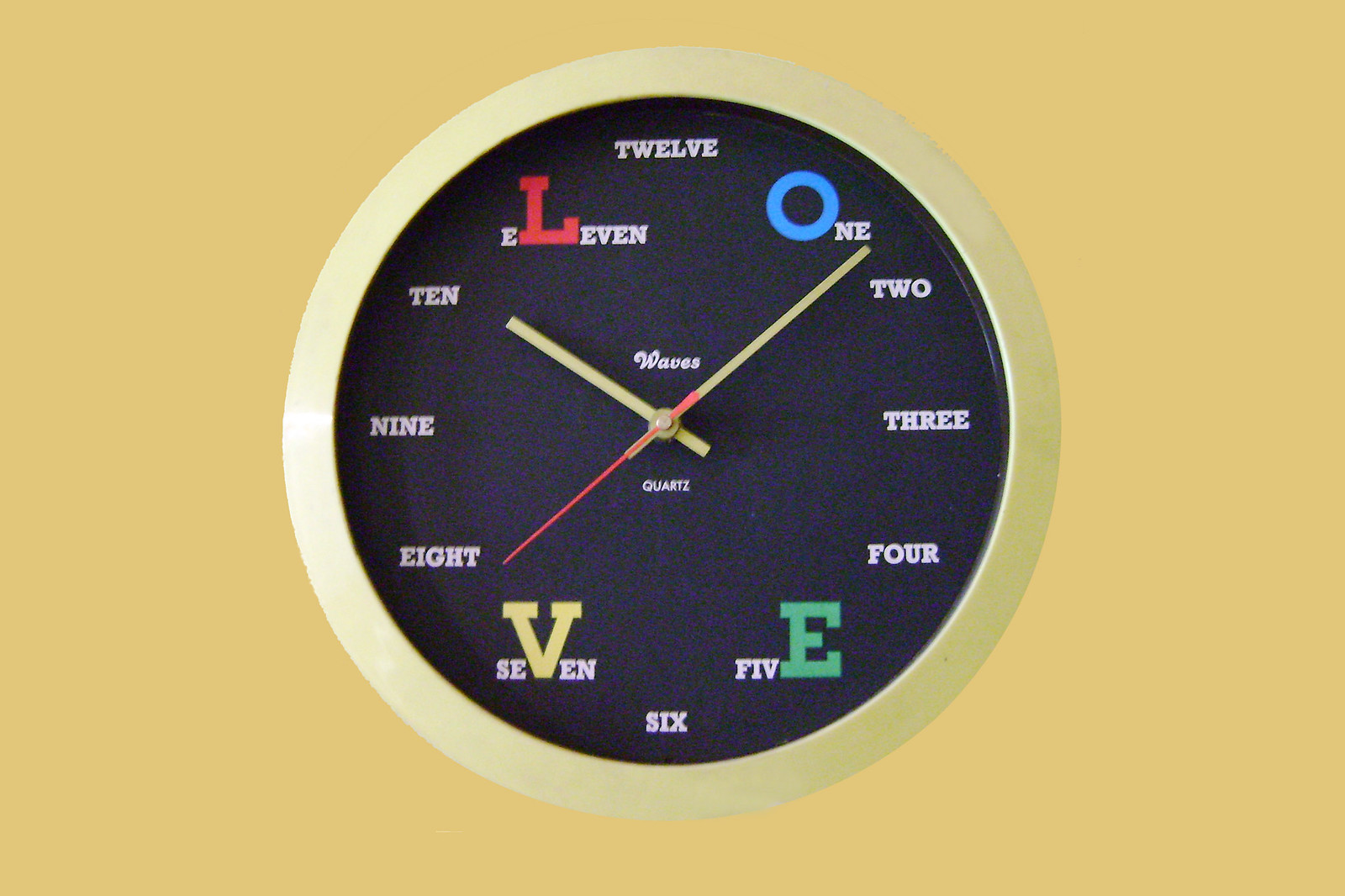This photograph features a unique, circular wall clock with a white or mustard yellow trim. The clock face itself is deep navy blue or black, possibly with a velvety texture, creating a striking contrast against the trim. Instead of traditional numerals, the hours are fully spelled out in white text, from "one" at 1 o'clock to "twelve" at 12 o'clock. Notably, certain letters in the numbers are emphasized and color-coded to spell out the word "LOVE." Clockwise, the bold letters form an 'L' in "eleven" at the top in red, an 'O' in "one" on the right in blue, a 'V' in "seven" at the bottom left in yellow, and an 'E' in "five" at the bottom right in green. The clock hands are ivory or gold in color, with the second hand standing out in red. In the center, the words "Waves" and "Quartz" can be seen, potentially indicating the clock's brand or model. Despite its classic analog display, the clock's creative design captivates with its colorful and meaningful presentation.